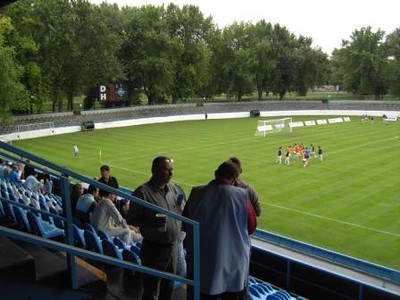This photograph, taken from the stands of an outdoor soccer stadium, captures a broad view of the scene. In the foreground, a trio of individuals stands on a stairway at the lower middle part of the image. One person, clad in a blue raincoat, has their back to the camera, while two others face them. Adjacent to this stairway is a blue handrail that stretches upward towards the left side of the image.

Surrounding them are rows of blue seats, mostly empty, though a few are occupied. To the right of the group, additional seats are visible with a rail running in front of them. Beyond the seats, the soccer field spans the middle portion of the image, featuring a prominent soccer goal. Players, dressed in red and blue uniforms, cluster near the right center of the field, seemingly preparing for a game or practice.

Encircling the field is a short white barrier, and farther out, there’s a larger gray fence. The background of the image is dominated by a grove of trees, with a bit of sky visible at the top right, characterized by a white expanse. Notably, a black sign with the letters "DH" and some indistinct images looms in the distance.